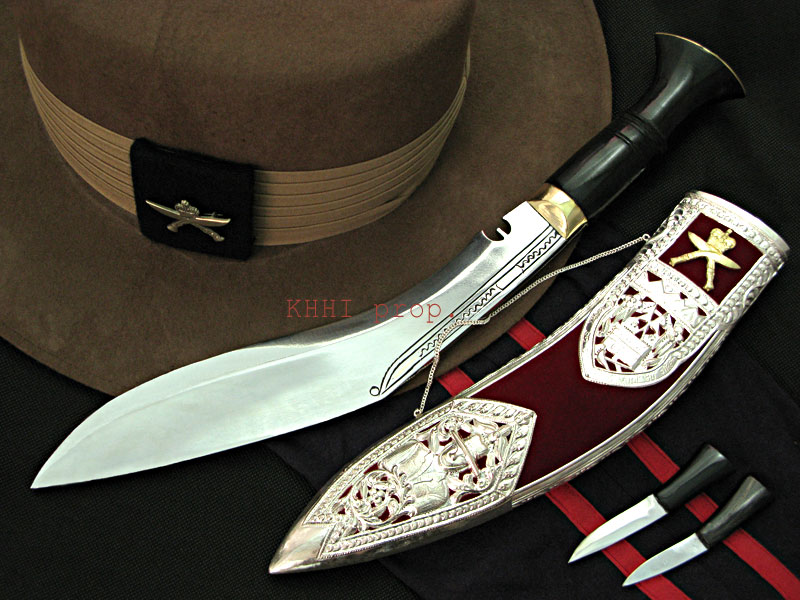The image presents a highly detailed scene featuring a brown sheriff's hat adorned with a strap and a pin showcasing a pair of crossed knives. Accompanying the hat is a prominent knife resembling a machete or small sword, with an intricately engraved curved blade and a black handle embellished with gold trim. The knife's ornate sheath is covered in luxurious red velvet cloth with intricate silver floral designs and chrome accents, adding a touch of royal elegance. Adjacent to the sheath are two smaller matching daggers, all placed on what appears to be a uniform or piece of black cloth with two red stripes. Faint text in the center of the image reads "KHHI Props," suggesting that these items might be movie props, with cohesive elements symbolized by matching symbols on the knife sheath and the hat's pin.